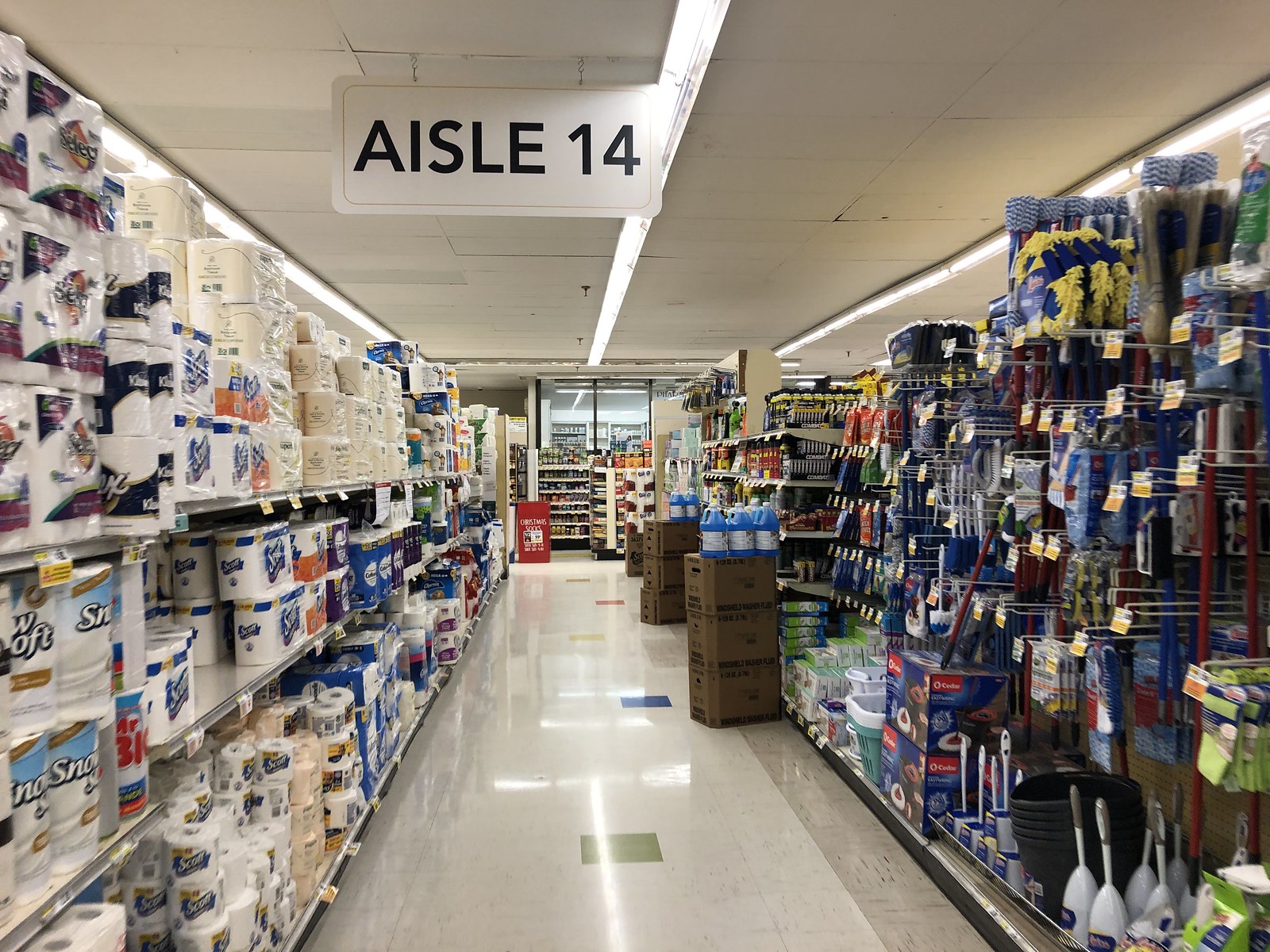The photograph captures the interior of a department store aisle crowned with a prominent Aisle 14 sign, suspended from a white acoustic tile ceiling illuminated by long white fluorescent lights. The floor is predominantly white linoleum, accented with a mosaic of decorative tiles in colors including green, blue, yellow, red, and gold, reflecting the lights above. To the left, three-tiered white shelves are stacked with various brands and types of paper towels and toilet paper. To the right, an array of household cleaning supplies is neatly organized, featuring items such as plungers, wastebaskets, toilet brushes, buckets, brooms, mops, and bottles of cleaning liquid. Among the cleaning supplies, dark brown cardboard boxes containing jugs filled with blue liquid and labeled with white stickers are visible. In the distance, the aisle leads to more white shelving units, possibly housing over-the-counter medications or other pharmacy goods, sheltered behind glass windows.